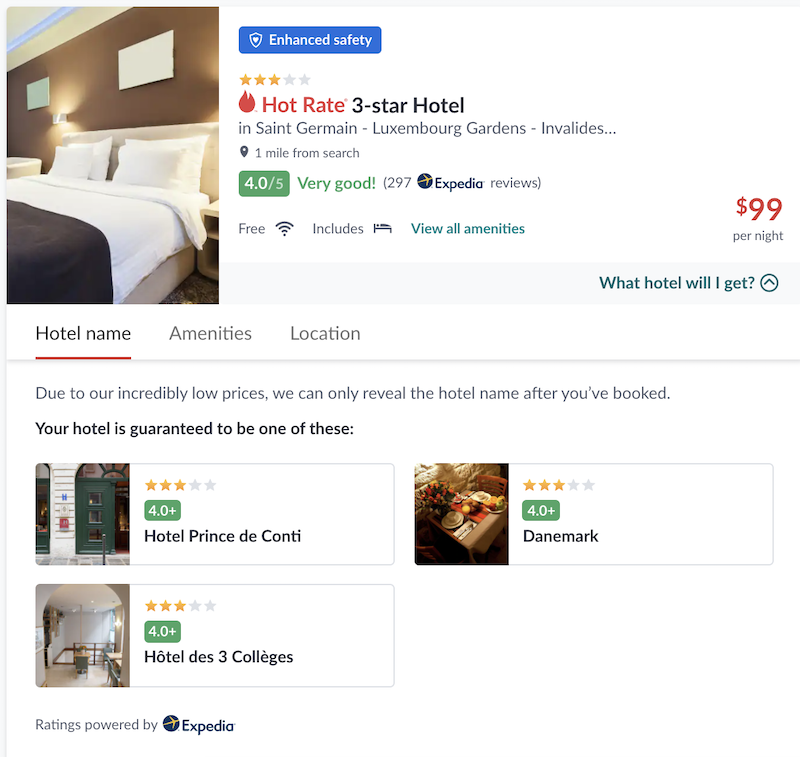This image is a screenshot from a travel website, with a white background, which seems to be associated with Expedia. There is no header visible at the top, but in the bottom left corner, a tiny "Ratings Powered by Expedia" text and the Expedia logo are present—a blue circle with a gold airplane and "Expedia" written in blue text.

At the upper left side of the screen, there is a photo showing a close-up of a hotel room. The bed is prominently displayed against a gold-colored wall and a very light beige headboard. To the right of this image, there is a blue rectangle with white text that reads "Enhanced Safety." The hotel has a three-star rating, illustrated by three gold stars and two gray ones. Below this rating, written in red with a small flame icon to the left, is the phrase "Hot Great." It also mentions "Three Star Hotel in St. Germain Luxembourg Garden."

On the right side of this section, the price is displayed in red as "$99 per night." Underneath, there is a note in black text stating, "Due to our incredibly low prices we can only reveal the hotel name after you've booked." This could indicate that the website might be a third-party platform using Expedia's content.

Additionally, the screenshot showcases three photos of different hotels. The first photo depicts an exterior view of a building in a city, shaded in blue. The second image (to the right of the first) is a close-up of a dining area, highlighting a well-set dining table adorned with flowers. The exact details of the food on the table remain indistinguishable due to the small size of the image.